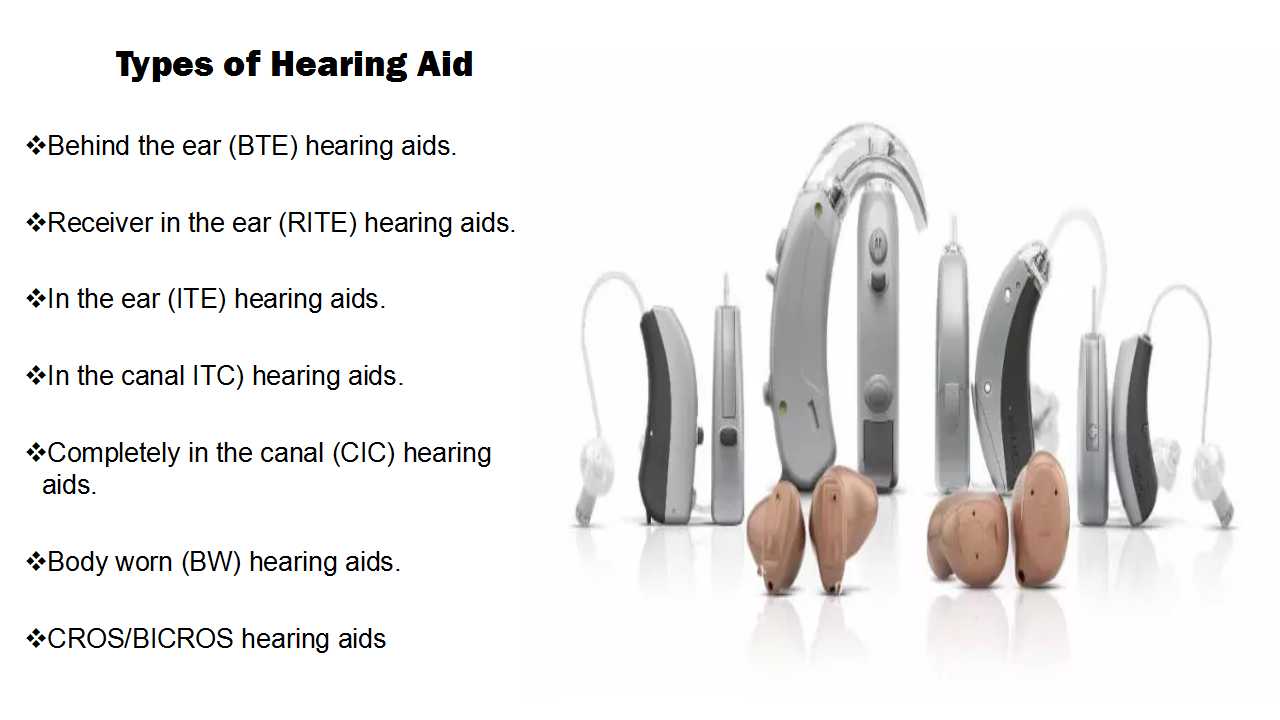This is an image for an advertisement promoting various types of hearing aids. The image is divided into two sections. On the left, in black text against a white background, it prominently reads "Types of Hearing Aid" followed by a list of different types in smaller, bulleted text: 

- Behind the Ear (BTE) hearing aids 
- Receiver in the Ear (RITE) hearing aids 
- In the Ear (ITE) hearing aids 
- In the Canal (ITC) hearing aids 
- Completely in the Canal (CIC) hearing aids 
- Body Worn (BW) hearing aids 
- CROS/BICROS hearing aids

On the right side, the image showcases photographs of various hearing aids, predominantly in silver and gray tones. These devices are slightly curved with larger components that appear to loop around the ear, with wires extending to smaller in-ear pieces. In front of these, there are four smaller, flesh-colored hearing aids, arranged in two pairs, designed to be more discreet and blend with skin tones.